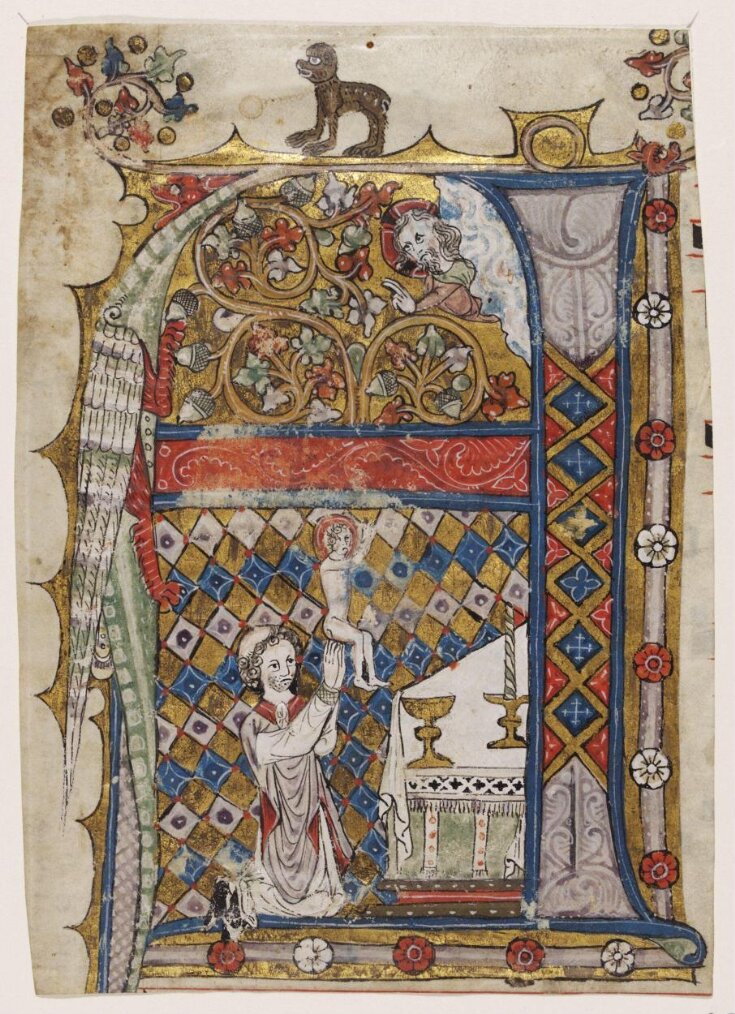The image in question appears to be a detailed photograph of an ancient, medieval fresco or mural, possibly dating back to the early Middle Ages (900s-1000s). It depicts a religious, Christian scene that seems to come from a church setting, resembling the stylistic elements of religious manuscripts from that era. 

In the foreground, there is a kneeling man, likely a saint or monk, with a bald head and a fringe of curly hair. He is dressed in a white robe accented with red, and he holds up a baby Jesus, identifiable by the halo around the child’s head. The saint’s hands are together in a prayer-like position. 

To his side is an altar adorned with gold candlesticks and a striped candle. The background reveals a checkered pattern motif of gold, blue, and white, resembling a canopy enclosure decorated with red and white floral designs. Floating above the altar, amidst some clouds, is the head of another man with a halo, likely representing God or another holy figure, watching over the scene.

At the top of the fresco, perched on the canopy, is a strangely depicted animal-like figure, which resembles a dog. Alongside this creature, there is a branch with birds, adding an additional layer of intricate detail to this historic artwork. The overall color palette includes dark red, blue, and gold, enhancing the solemn yet regal atmosphere of the depiction.